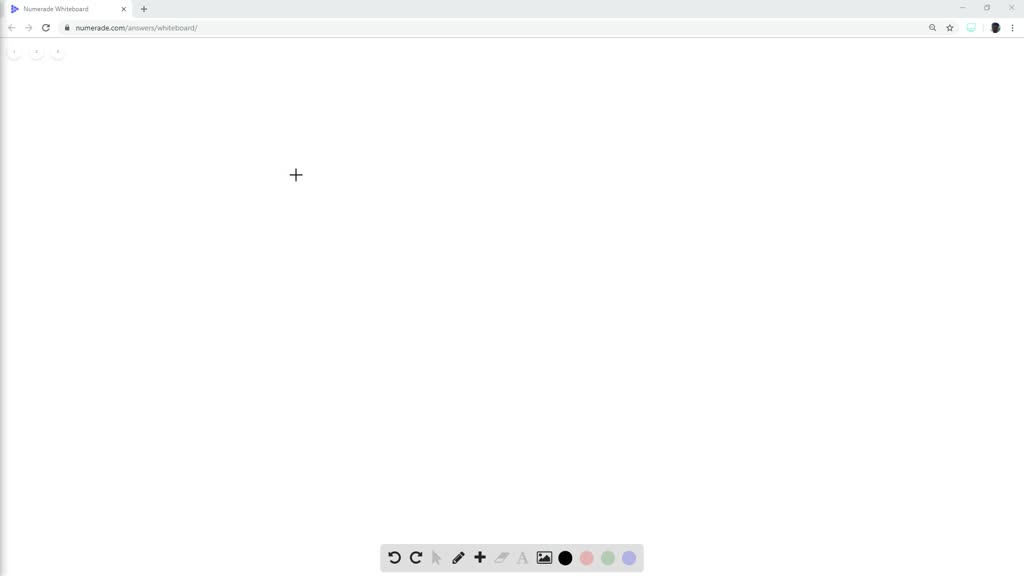In this screenshot, we primarily observe a user interface dominated by white space, organized as follows:

At the top, there's a mid-grey bezel that contains several elements. On the far left, a white tab is present, housing a triangular logo fashioned from multiple purple circles, which is tilted to the right. Accompanying this logo is grey text that reads "NumerAD Whiteboard" (spelled as N-U-M-E-R-A-D). Directly beside it, there’s a black 'X' icon.

Adjacent to these, a black cross icon is visible, intended for adding new tabs. Additionally, there is a set of grey navigational arrows; one pointing to the left and the other to the right, coupled with a black refresh symbol. An oval-shaped URL display featuring a black lock symbol is included, indicating a secure connection. Next to the lock, the black text reads "numerad.com."

The URL is followed by a grey backslash trail that reads "/answers/whiteboard/". On the right side of the bezel, a dark grey magnifying glass icon and a similarly colored star icon are present. Further to the right, three control icons— a minus, two overlaid squares, and a close 'X'— are visible on the bezel's far-right end. Next to them, there's a teal silhouette of a computer, a user profile picture, and three vertically aligned black ellipses.

Beneath the bezel, a vast white area serves as the main workspace. Embedded within this space are three small, white circles labeled "1", "2", and "3" in black. A black crosshair cursor is centered on the screen.

At the bottom, a dark grey floating rectangle hosts several tools and options. These include a left-curving black undo symbol, a right-curving black redo symbol, a grey pointer, a black pencil, a black cross, a grey paintbrush, and a capital 'A' in grey. Further along the toolset, a black icon of a square with mountains and a sun, symbolizing importing a picture or a screenshot, can be seen. The final elements of this toolbar are a sequence of colored circles: black, purple, green, and another purple circle.